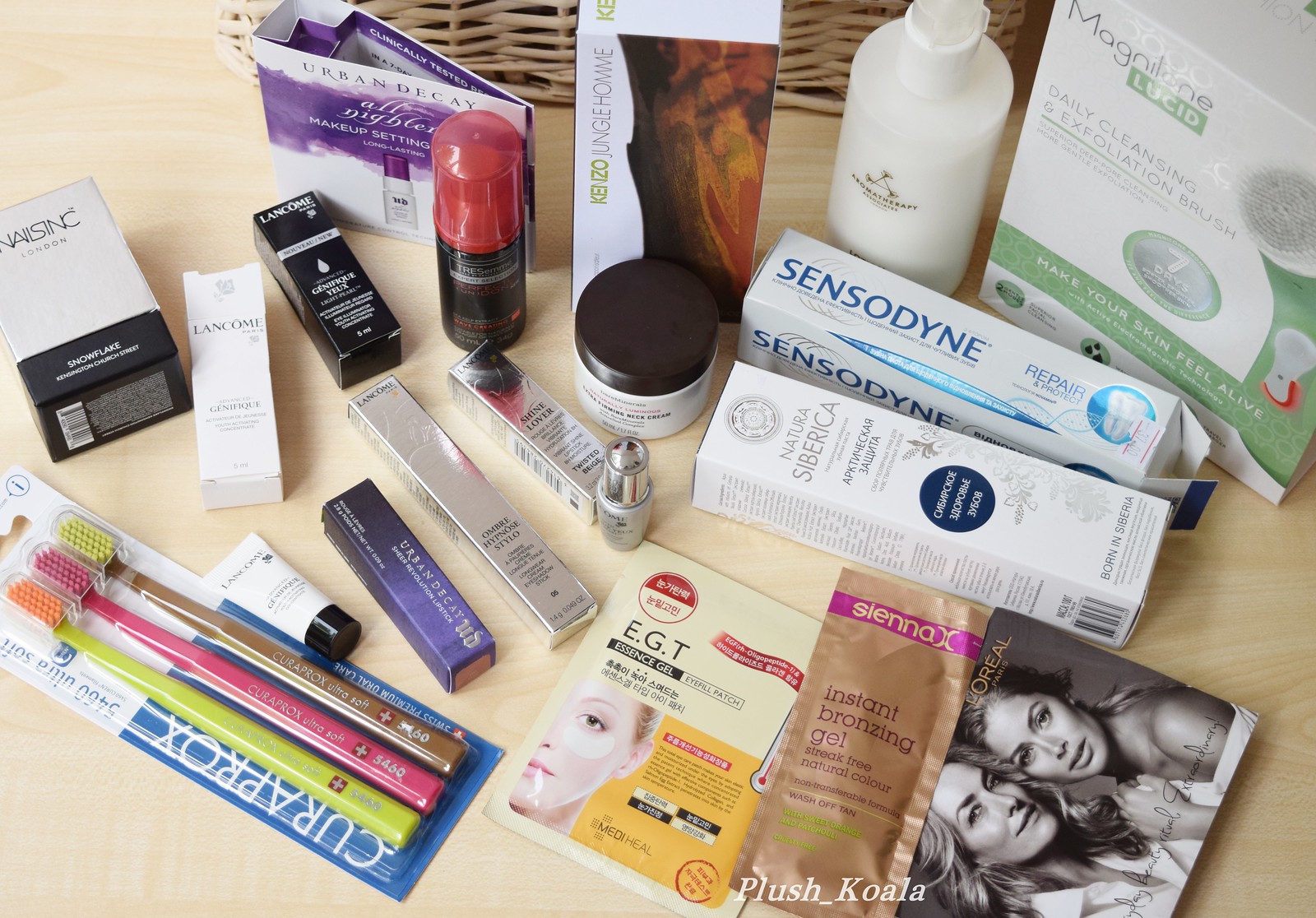In the image, we observe an assortment of items from a shopping haul laid out on a light oak-colored desk, slightly off-center towards the right. The desk displays the name "plush_koala" typed at the bottom. Among the various hygiene products, there's a wicker basket in the background. The haul includes several brushes, a tube of instant bronzing gel, and Sensodyne toothpaste—all of which are travel or sample-sized products. We also notice a facial spin brush in a box labeled "Magna Line Lucid Daily Cleansing and Exfoliation Brush - Make Your Skin Feel Alive." Additionally, the collection includes different makeup samples from brands like Lancôme, NutraTabera, L'Oréal Paris, and EGT.